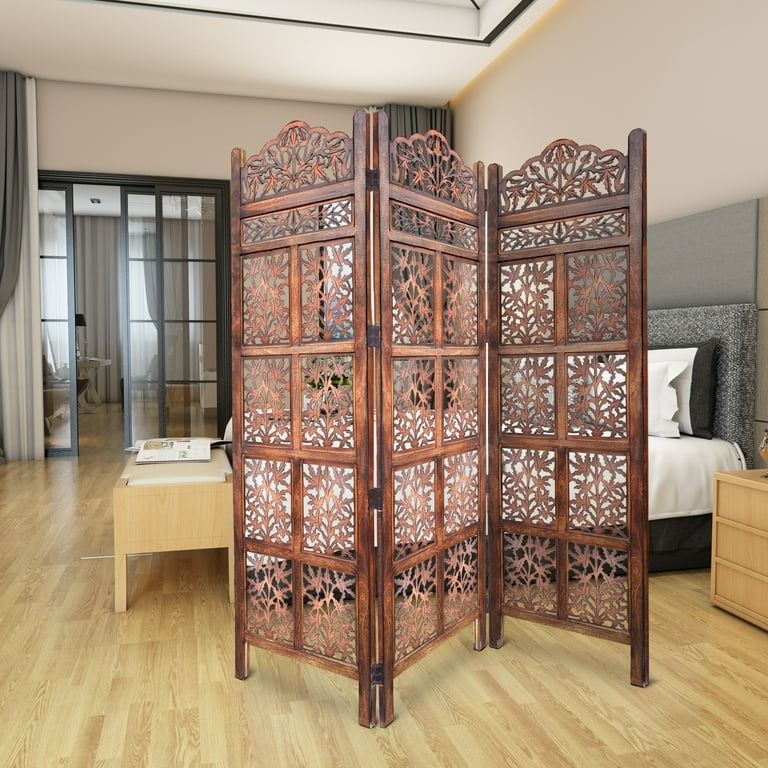The image is a detailed photograph of a modern bedroom with a light tan hardwood floor. The camera captures a vertical, rectangular view that includes a tall, ornate wooden room separator at the forefront. This three-section, latticed screen with arched tops partially obscures the bed behind it. The bed, positioned against a light gray wall, features a large gray cloth headboard, with pillows propped up against it. A small table at the foot of the bed holds an open book.

On the right side of the image, there is a bedside stand with three drawers, also in the light wood that matches the floor. A set of glass-paneled double doors is located near the left edge of the picture; these doors are flanked by white drapes and slide open to reveal another room. Additionally, the roof above the bed is recessed and bordered in green, adding to the modern aesthetic of this thoughtfully designed space.